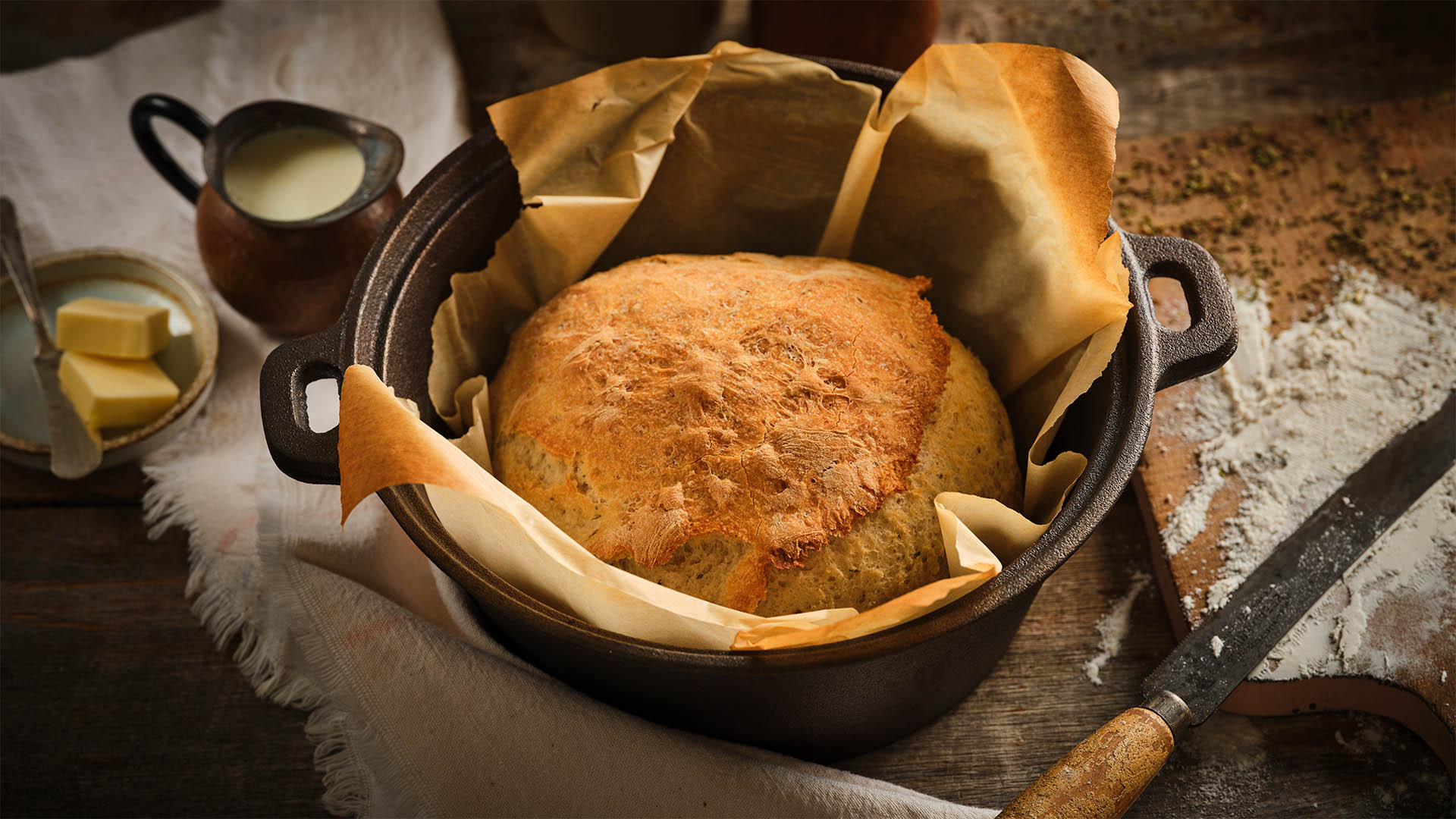The image features a freshly baked round loaf of sourdough bread nestled in a black cast iron pot lined with parchment paper, the bread’s golden-brown crust contrasting the dark vessel. To the left of the pot, there is a small butter dish holding two thick pads of butter and a butter knife resting alongside it. Adjacent to the butter dish is a petite copper pitcher with a metal handle, containing a whitish liquid that could be milk, cream, or possibly cheese. On the right side, a light brown wooden cutting board dusted with flour and a mix of spices is laid out. A knife featuring a round wooden handle is placed diagonally across the board. Beneath all these items lies a white linen tablecloth with tassels at the edges, spread over a dark brown wooden table, tying together the warm and rustic scene.